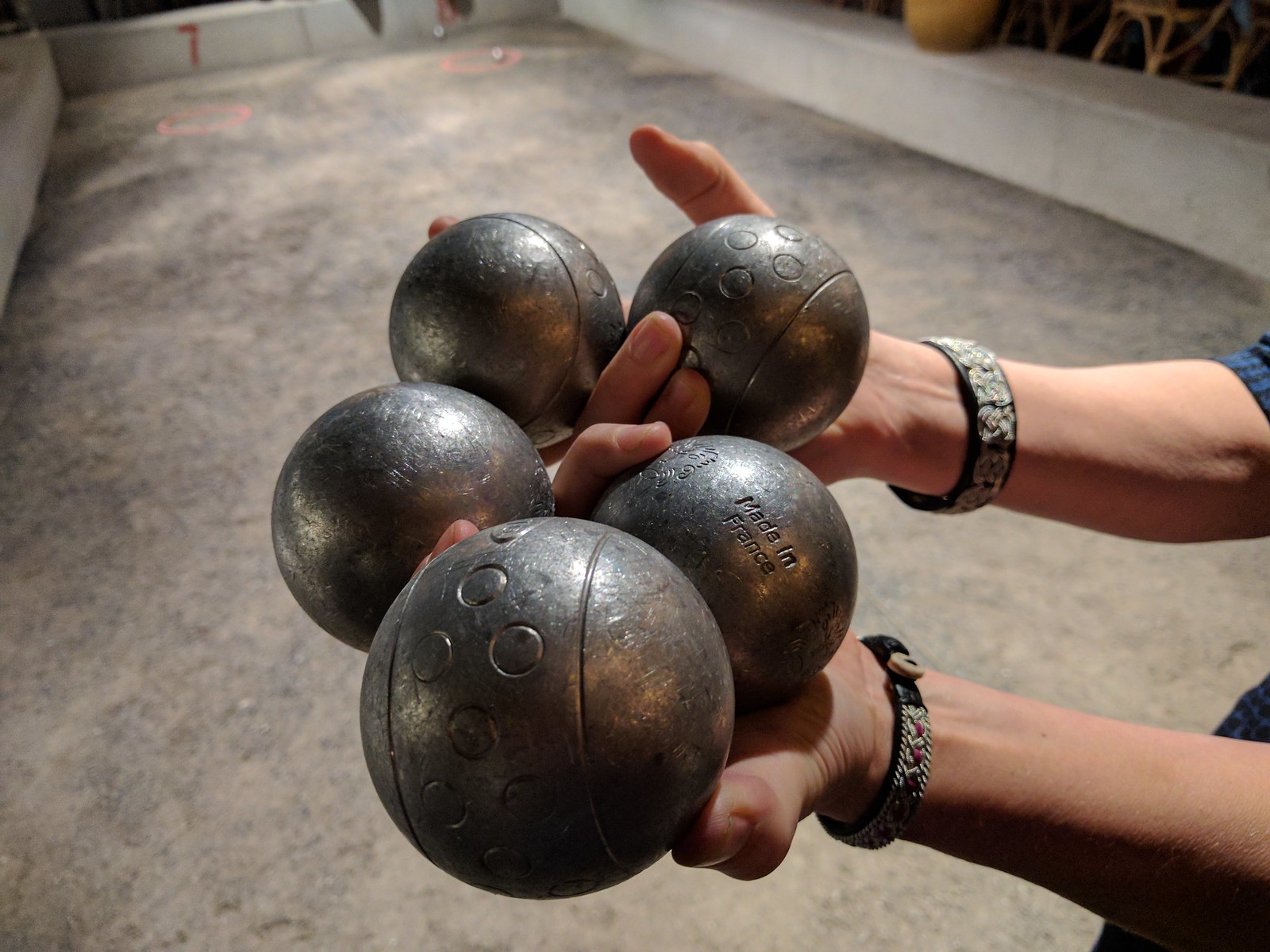In this rectangular photograph, we see a person’s forearms, palms up, extending from the right side of the image towards the left. The person's arms are adorned with leather bracelets on their wrists, and they are wearing a blue shirt. Holding between their fingers are five engraved metal balls of varying sizes, with the largest ball positioned at the lower center. Each ball features an intricate pattern of engraved circles and bands around its circumference. One of the balls on the lower right is clearly engraved with the words "Made in France." The balls appear heavy and could possibly be weights or cannonballs. The background, which hints at a beige, creamy marble or bowling area, remains nondescript, providing no additional context for the location. Despite this, the detailed focus on the hands and the metal balls captures a scene of strength and intricate craftsmanship.